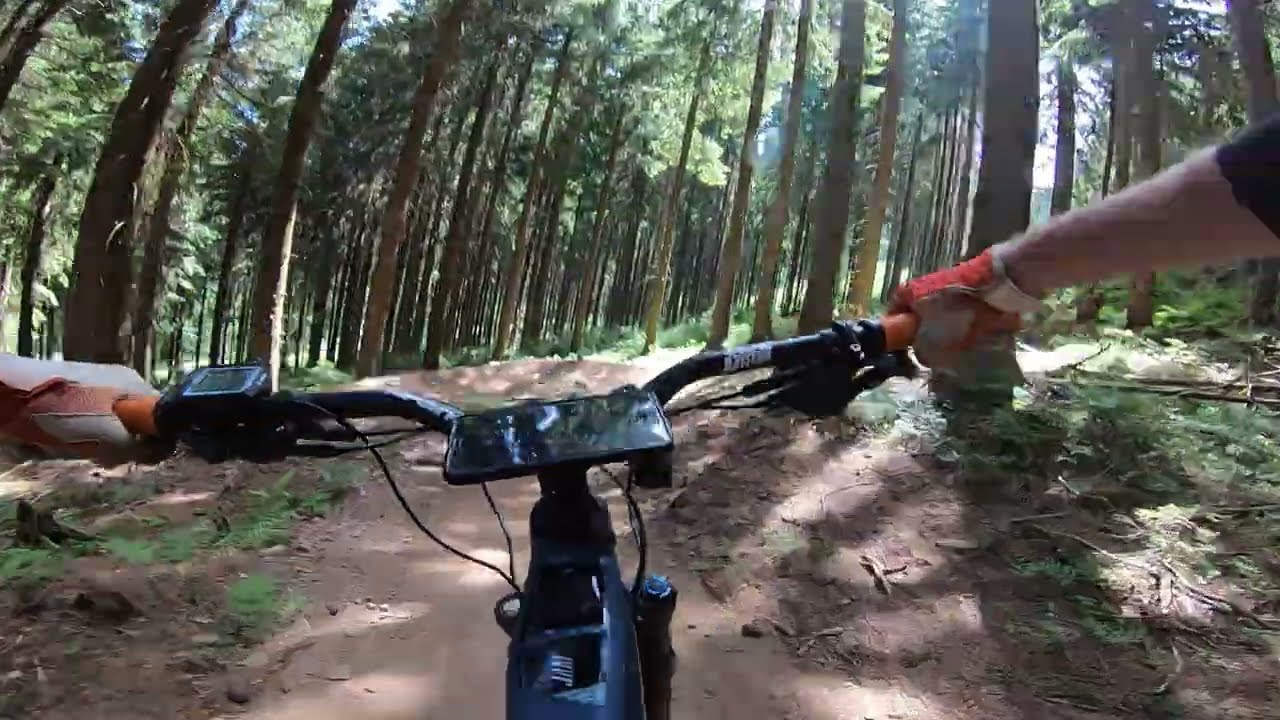The photograph captures the exhilarating perspective of a mountain biker navigating a rugged dirt trail deep within a dense forest, likely taken from a GoPro mounted on their chest. The biker's white-skinned hands, wrapped in tan and orange gloves, grip the handlebars firmly. Centered on the handlebars is a phone, miraculously balanced within its mount, while a square speedometer or tracker sits on the left side, its wire trailing down towards the wheels, indicating the miles traveled. As the trail ascends and twists to the left, it vanishes into the thick woodland. Lush ferns and sparse shrubs line the path, while towering evergreen trees, devoid of low branches, stretch upwards, their trunks bathed in dappled sunlight filtering through the canopy. The scene is a majestic interplay of nature and adventure, captured from the rider's dynamic vantage point.